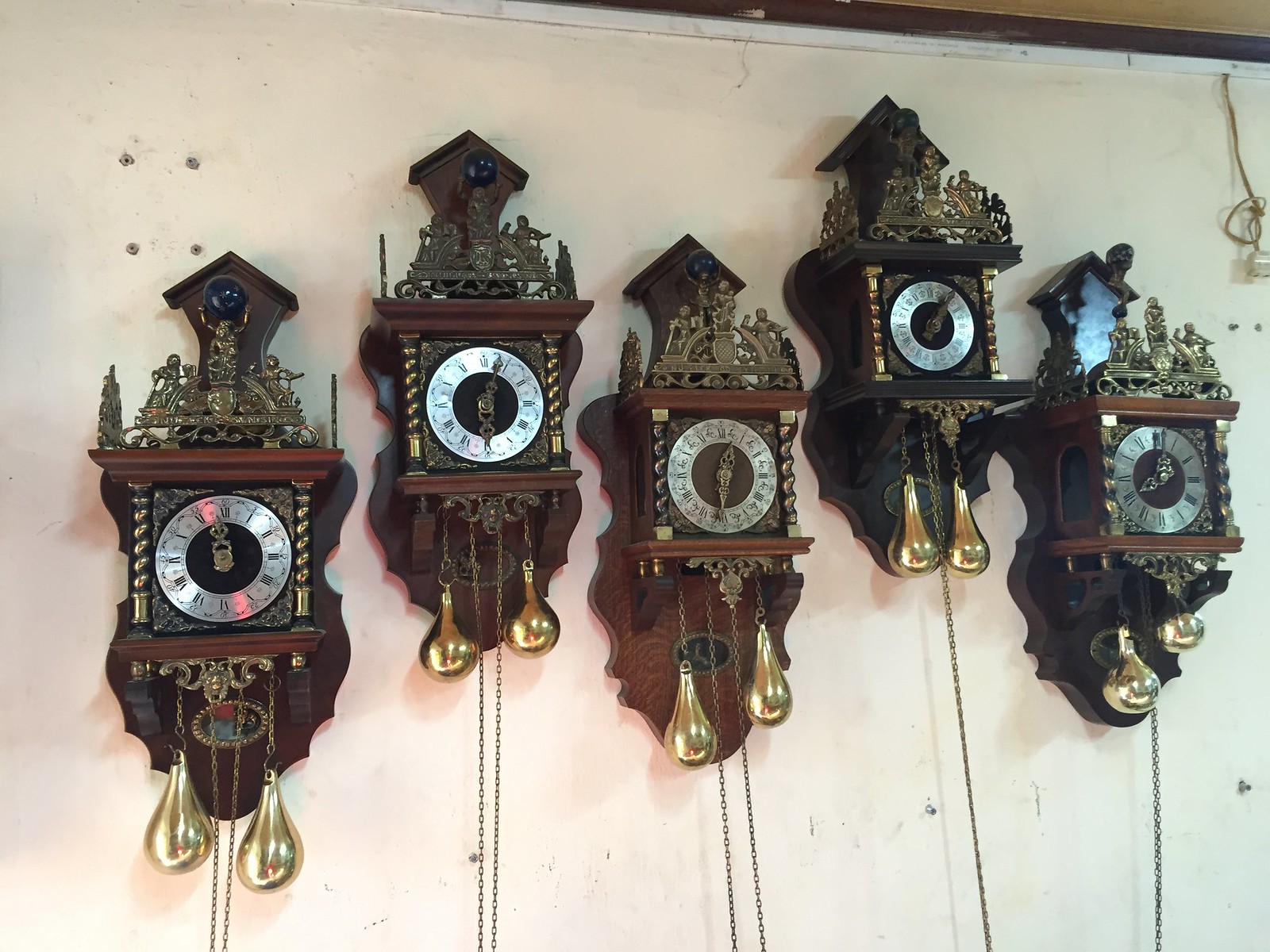This image showcases a collection of five intricately designed cuckoo clocks, all hanging on a wall. Each clock is adorned with elaborate carvings and decorations. These clocks vary in color, with three made of brown wood—ranging from light to medium shades—and two crafted from dark, almost black wood. Every clock features a pair of gold balls hanging at the bottom, connected by two chain link ropes, which add to their ornate appearance.

At the top of each clock, there's a brass or golden decorative element resembling a tiara or crown. This decoration typically includes two human figures standing on either side, holding objects in their hands, with a prominent figure in the center holding a blue ball above their head. However, variations exist, such as one clock where the central figure is holding a harp instead.

The times displayed on the clocks vary, with the first clock showing nearly 12:00, the second and third clocks indicating 12:30 with slight differences in their decorations, the fourth clock reading 1:05, and the fifth clock depicting around 7:00 or 8:00. The faces of the clocks are silver with ornate metal dials and winding spiral columns on either side, showcasing the craftsmanship involved in their creation. The detailed gold and silver elements, combined with the dark and brown woods, create a visually striking and cohesive display of timepieces.